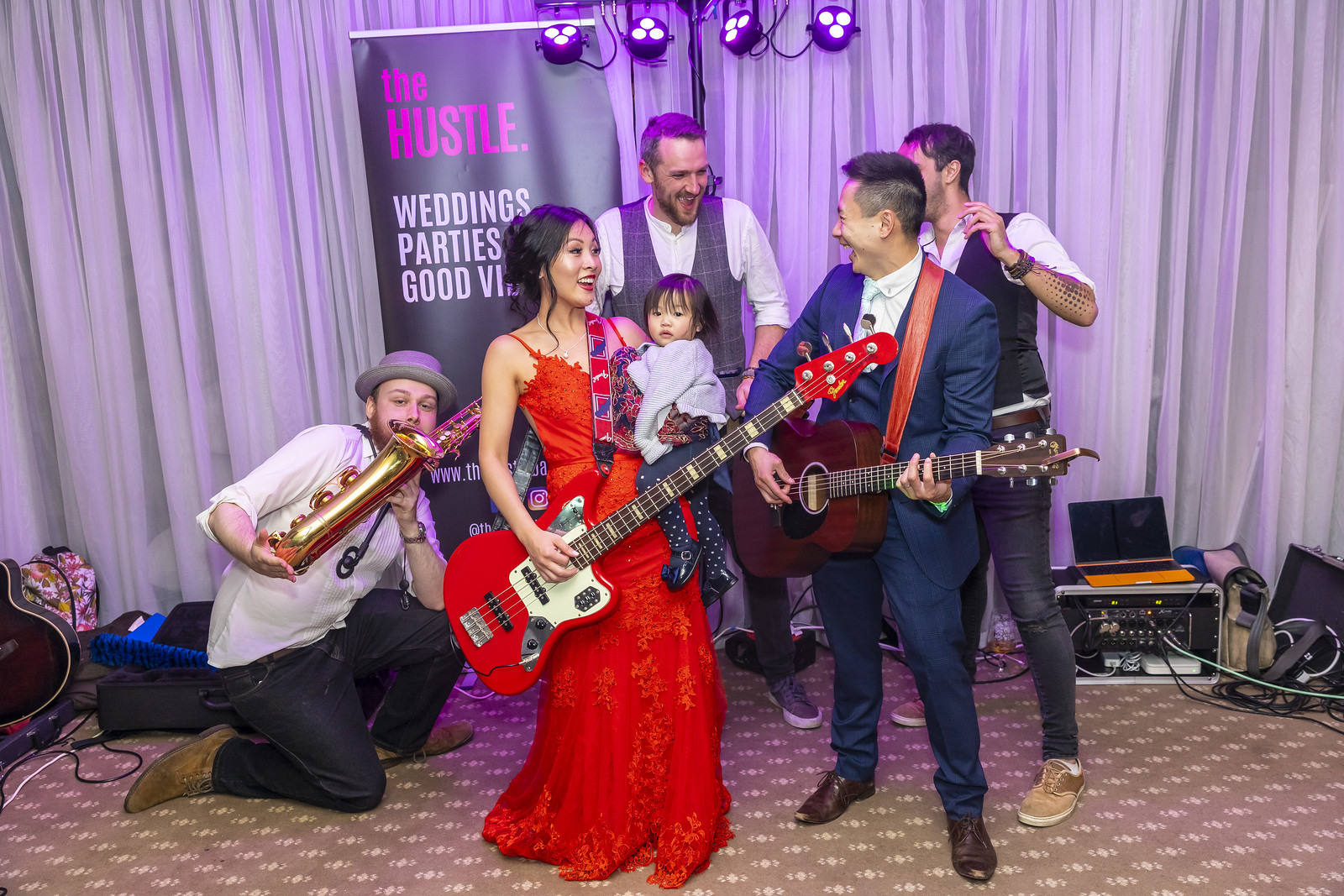The photo captures a lively group that appears to be a band, standing in front of a light purple curtain adorned with a sign reading, "The Hustle, Wedding Parties, Good Vibes." The atmosphere is vibrant, with everyone grinning and seemingly preparing for a performance. Central to the image is an Asian woman in a long red dress holding both a red electric guitar and a small infant dressed in blue and white polka dot tights. She is joined by a man to her right, kneeling and playing a tenor saxophone, dressed in a white shirt. On her left stands another man, wearing a blue suit and holding an acoustic guitar, glancing at her with a broad smile. Behind this trio are two more men: one dressed in a vest and long sleeve dress shirt and the other partially obscured. The backdrop features various musical equipment scattered around, while they stand on a printed tan and white rug. The diverse group, possibly Hispanic or Asian, exudes joy and excitement as they ready themselves, creating an atmosphere brimming with good vibes and the promise of engaging music.